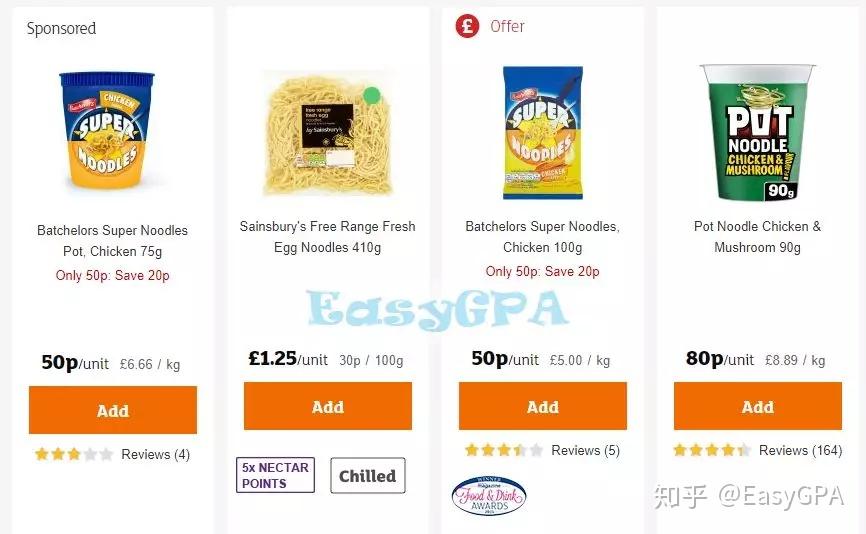The screenshot displays a promotional section from a website showcasing different food products under the "Sponsored" label in the upper left corner. The featured items include:

1. **Bachelor's Super Noodles Pot Chicken, 75 grams** - Priced at 50p with a savings of 20p off the original price, making it 50p per unit.
2. **Sainsbury's Free Range Fresh Egg Noodles, 410 grams** - Priced at £1.25 per unit.
3. **Bachelor's Super Noodles Chicken, 100 grams** - Priced at 50p with a savings of 20p off the original price, making it 50p per unit.
4. **Pot Noodle Chicken and Mushroom, 90 grams** - Priced at 80p per unit.

Each product listing is accompanied by an orange "Add" button, likely for adding the items to an online shopping cart.